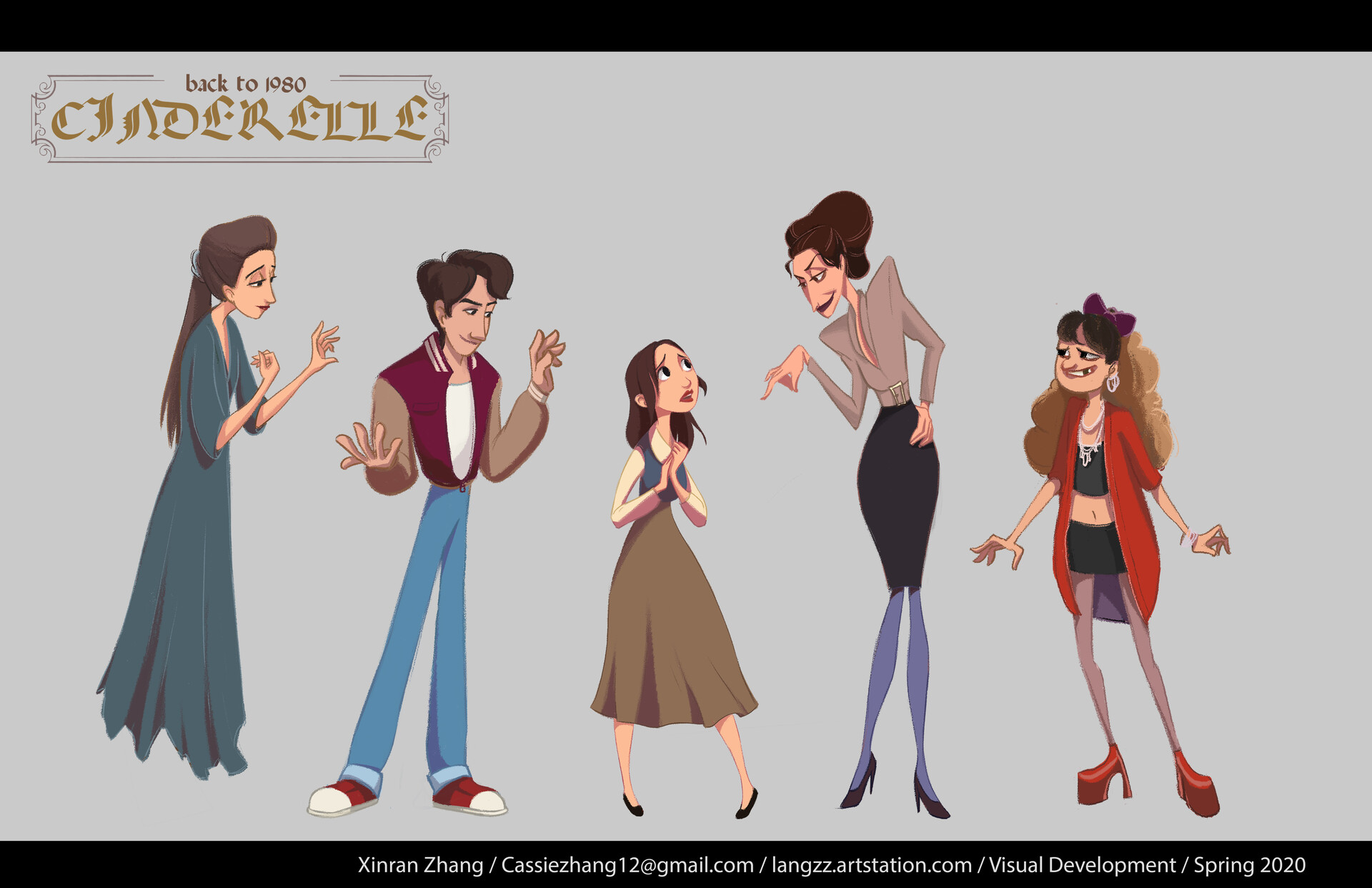In the center of the image, five cartoon characters stand against a gray background trimmed with black at the top and bottom. The characters, predominantly female, appear lively and distinct.

On the far left, a woman in a long, jagged-hemmed blue dress seems to be slightly elevated, her shoes not visible. She has long brown hair tied in a ponytail and extends her arms while gazing at the man to the right.

Next to her stands the only male character, dressed in blue jeans, red and white shoes, a brown and red jacket, and a white t-shirt. His brown hair complements his look, and he has his arms raised with elbows bent, directing his attention to the female character in the middle.

The middle character, significantly shorter, sports black shoes and a brown dress that falls just below her knees. She wears a white shirt underneath a blue vest and looks up at the woman to her right with a rather fearful expression. Her hands are clasped together near her chest, elbows bent.

To her right, another female character is dressed in a tight brown blouse with pointed shoulders and a black skirt. She has short brown hair and wears blue-purple stockings with black high heels. Pointing at the middle character, she stands with conviction.

The fifth and final character on the far right wears a black jacket reaching just above her knees, paired with red heels, a black crop top, and a very short black skirt. Her long blondish-brown hair flows freely, and she displays a smile. With her arms slightly extended outward, her hands are open. Adorning dark earrings and a bow, she exudes confidence.

In the upper right corner, text reads, "Back to 1980," with "Cinderella" elegantly framed beneath it. At the bottom of the image, contact and portfolio information is provided: "xingrangzang/cassieshang12@gmail.com/langs2zs.artstation.com/visualdevelopment/spring2020."